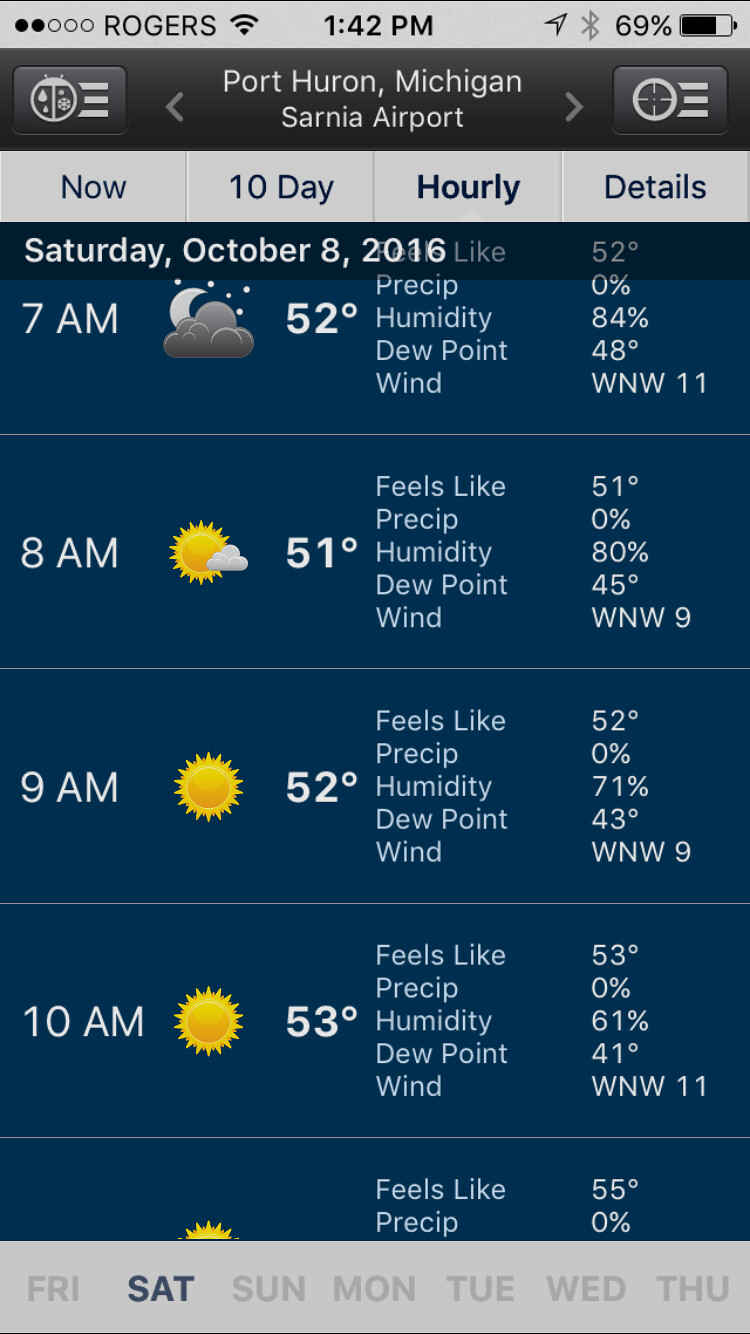This is a detailed screenshot of a weather forecast app on a mobile device, likely an iOS device given the top bar details. It shows Port Huron, Michigan, Sarnia Airport, and features several viewing options like "Now," "10 Days," "Hourly," and "Details," with the "Hourly" tab selected. The date is Saturday, October 8, 2016, and the highlighted day at the bottom confirms it is Saturday. The hourly forecast provides specific weather details from 7 AM to 10 AM, including temperatures of 52°F at 7 AM, 51°F at 8 AM, 52°F at 9 AM, and 53°F at 10 AM. Weather conditions show partly cloudy at 7 AM and 8 AM, with sunny conditions from 9 AM to 10 AM. Additional weather metrics include 0% precipitation, 84% humidity, a dew point of 48°F, and winds from the west-northwest at 11 mph. The device status bar shows it is 1:42 PM with 69% battery remaining, Wi-Fi connected, and low signal strength on the Rogers network.